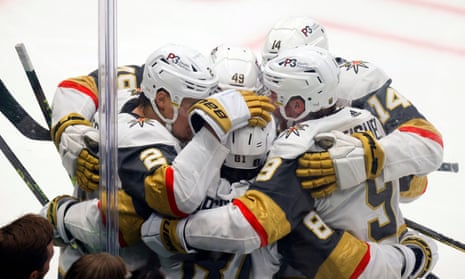An angled view captures a huddle of five male hockey players embracing in celebration on an ice rink. Their white uniforms feature blue, yellow, and red stripes on the sleeves, and they wear white helmets and yellow gloves. Visible numbers on the jerseys include 14, 9, 8, and 2, while the helmets display numbers like 49 and P3. Some players' hands rest on their teammates' helmets, while hockey sticks jut out from the sides of the group. The background reveals the icy rink with red lines bisecting it, and in the lower left corner, spectators' heads are seen behind the protective glass, witnessing the moment of camaraderie and triumph.